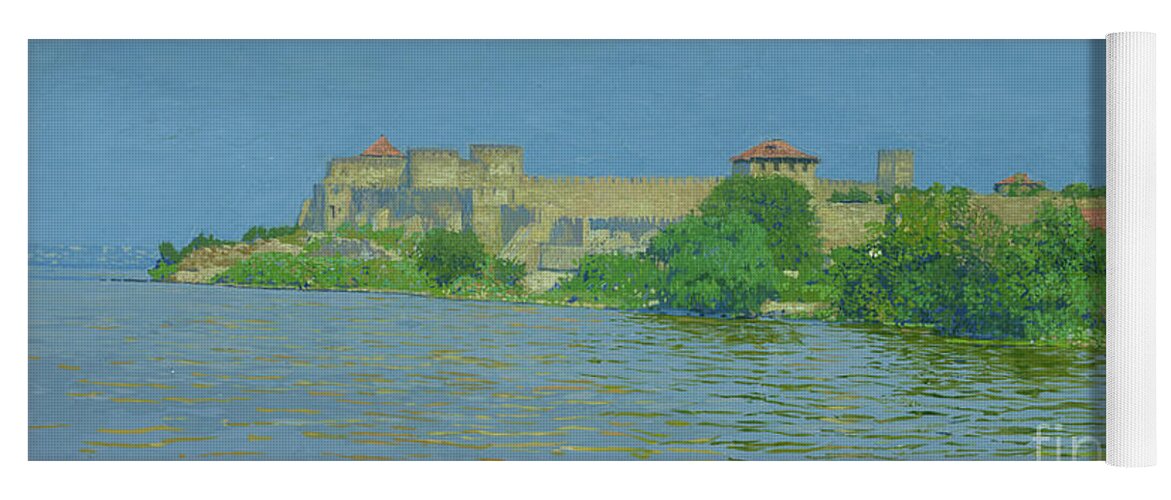The image depicts a finely detailed, realistic oil painting of a coastal seascape viewed across a body of water. Dominating the scene is a large stone fortress with numerous turrets, some of which are topped with rust-colored, terracotta roofs, while others are roofless. Set upon a lush, green peninsula with thick shrubs and large bushes, the fortress' stonework varies in hues of light and dark beige. The expansive, rippling water extends to meet the horizon on the left, while the sky above is a clear blue, nearly blending with the water's color. To the right side of the image, where the painting seems to suggest it could be rolled like a scroll, additional structures with red and flat roofs are visible along the water's edge, all contributing to the tranquil yet grandiose coastal landscape.